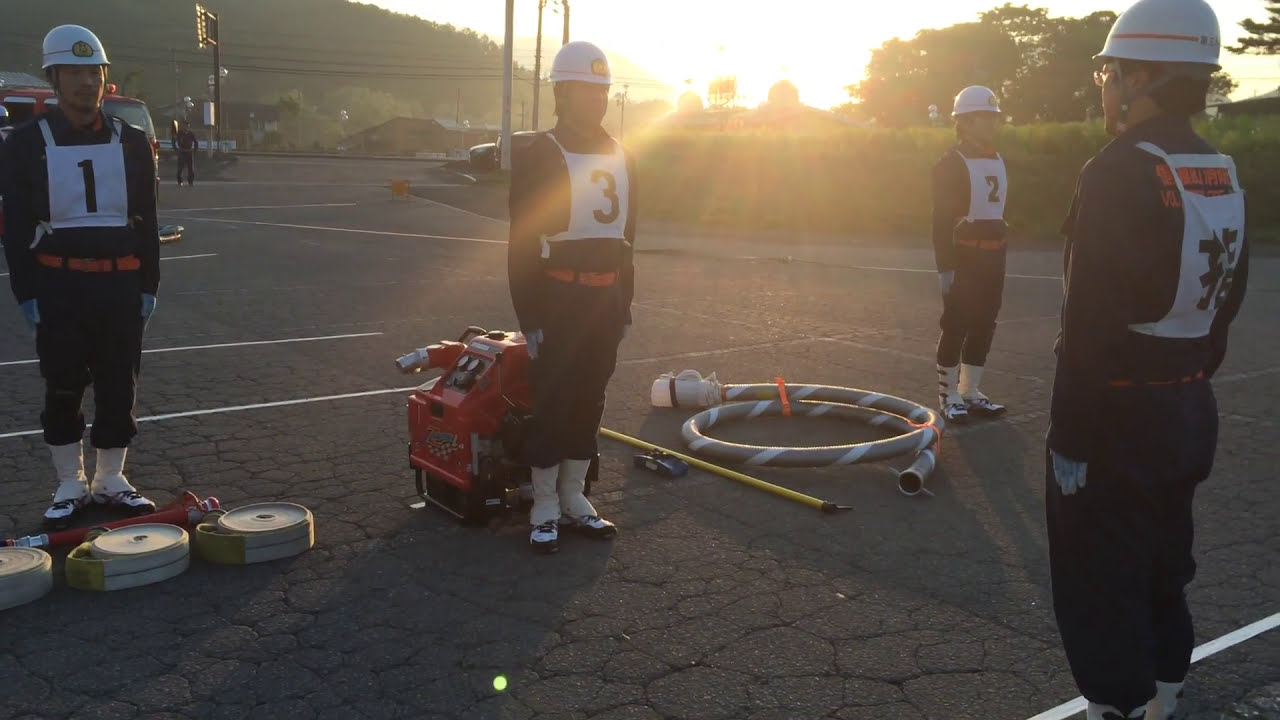This photograph captures a field training exercise against a verdant outdoor backdrop. In the image, four Asian men are dressed in matching black uniforms with white socks and black sneakers. Each man also wears a bib featuring a number: 1, 3, or 2, except for the fourth man whose bib displays an Asian character on the back. The man with the character is positioned in the bottom right corner, addressing the other three men who stand at attention. Various objects lie on the ground around them, including three canisters in front of the man numbered 1, a coil of wire or cable between the men numbered 2 and 3, and a red generator behind the man in the middle. The setting features a cracked, green pavement with white lines, and in the background, a picturesque hill covered in trees is illuminated by the bright sunlight.